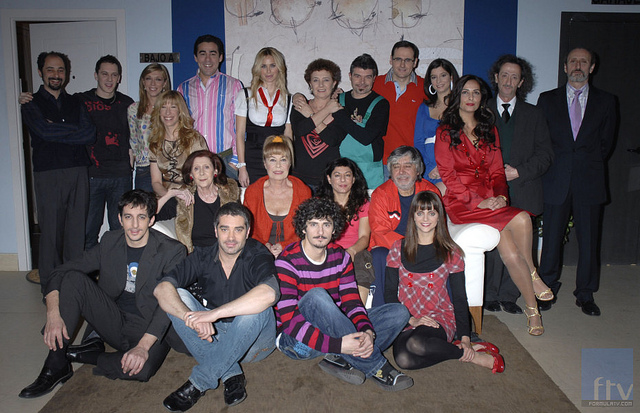This image captures a diverse group photo of approximately 20 people, arranged in three distinct rows, suggesting a company staff gathering or special event, possibly a holiday party. The back row features individuals standing, predominantly in formal attire such as suits and a striking red dress. The middle row consists of people seated on a white couch, including an older demographic. The front row displays four individuals sitting on the floor, two of whom are wearing jeans, while others are in semi-formal or casual dress. The group is a mix of different age groups, comprising both men and women.

The setting appears to be indoors, within a building characterized by multi-colored walls; white walls flank either side, a navy blue section is in the middle, and a portion of the wall with peach or pink designs, albeit unclear, lies at the center. Contemporary art and possible scribbles add to the decor. There is a door visible on the left side with a sign that reads “Bajo A,” which could indicate a restroom. Another door is located at the right corner.

Additionally, there is a brown rug beneath the group on the floor, adding warmth to the scene. A small watermark with the logo "FTV," which stands for "Formula TV.com," is positioned in the bottom right corner of the image.